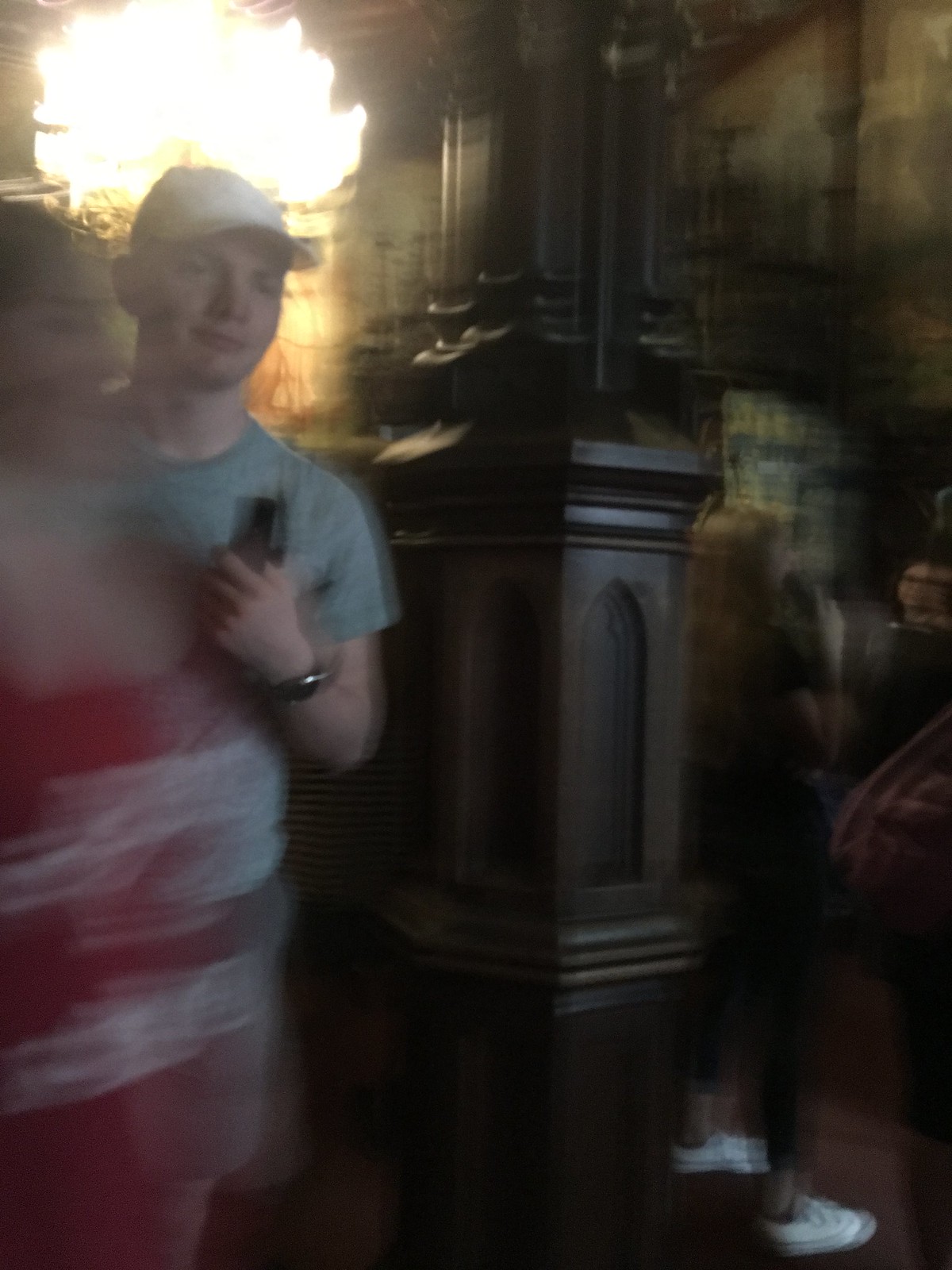A man in a gray shirt and white hat stands beside a beautifully crafted wooden pillar inside a church, likely a Catholic one judging by the architectural elements. In the background, the soft, warm light streaming through a window illuminates the space, casting a gentle glow on an array of wooden crucifixes depicting Jesus. The overall ambiance is serene, with blurred figures in the background adding to the sense of contemplative quietness.